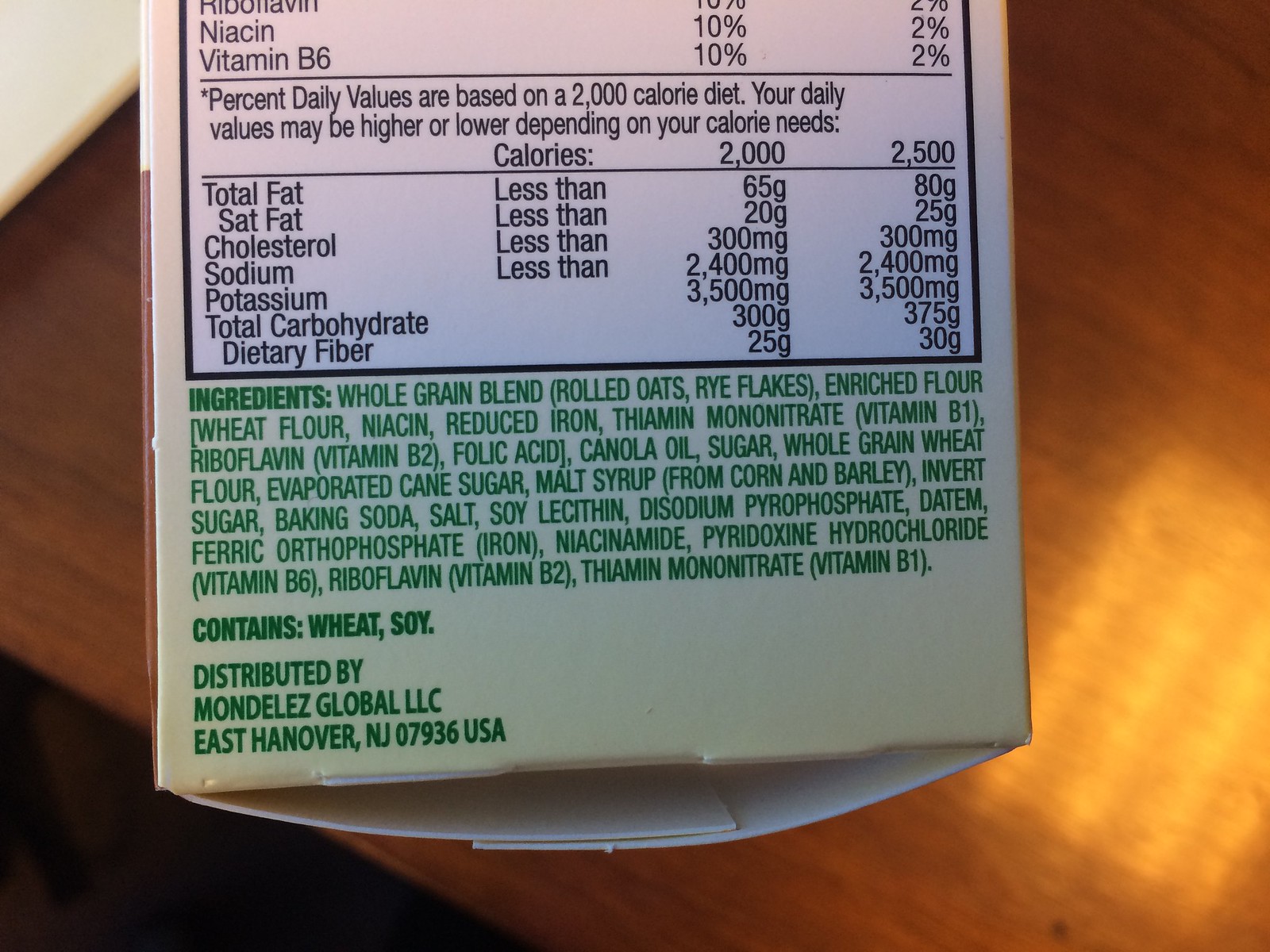The image displays a partial view of a cereal box's nutritional and ingredient information. The top section of the photo captures the nutritional facts, partially showing values like 10% Niacin and 10% Vitamin B6. Beneath this, the image reveals the full list of ingredients, written in green text. The ingredients list starts with a whole grain blend comprising rolled oats and rye flakes, followed by enriched flour, wheat flour, niacin, reduced iron, thiamin, and other nutrient additives. Additional components include cane sugar and malt syrup, indicating that the cereal has a sweet flavor profile. The label also notes that the product contains wheat and soy. The cereal is identified as being distributed by Mondelez Global, LLC, based in East Hanover, New Jersey.